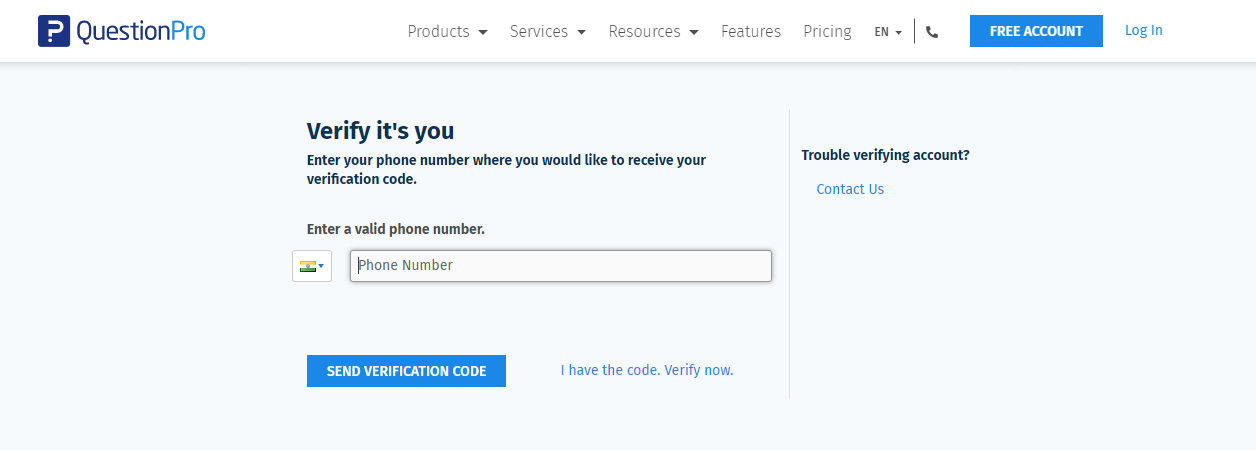Screenshot of the QuestionPro Verification Form:

In the upper left corner, the QuestionPro logo is prominently displayed, featuring a blue box with a question mark and the text "QuestionPro" beside it. The word "Question" is in a dark blue shade, while "Pro" is in a lighter blue. To the right of the logo, the navigation menu features several items in a row from left to right: Products, Services, Resources, Features, Pricing, and an option to change the language, currently set to English (indicated by the acronym "EN"). An icon of a telephone is situated next to the language setting.

Further to the right, there's a blue button with white text labeled "Free Account," followed by a blue text link for users to log in. Below the navigation menu, a prompt reads "Verify it's you," instructing users to enter their phone number for receiving a verification code. Beneath this instruction, smaller text advises to "enter a valid phone number." A text box is provided for the phone number entry. Below the text box, a blue button with white text prompts users to "Send Verification Code." To the right, a small blue text link offers an alternative option: "I have the code. Verify now."